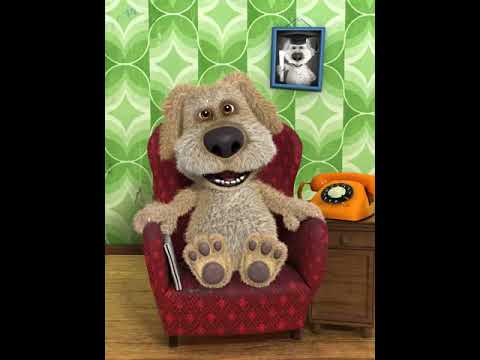The image is a detailed 3D graphic, depicting a somewhat scruffy, light brown dog with floppy ears and expressive brown eyes. The dog, which has a distinctive large, black oval-shaped nose and fuzzy hair surrounding it, is sitting in a red chair adorned with a lighter star or diamond pattern. Its front paws rest on the chair’s arms, and its back legs are visible, while its mouth is open showing its lower teeth. 

The setting includes a green wallpaper backdrop featuring diamond or star motifs and various stripes in a mix of light and dark green. Mounted on the wall to the upper right of the dog’s head is a blue-framed black and white picture of another dog, which appears to be wearing a graduation cap and holding a diploma. 

Next to the red chair is a small brown end table, which supports an old-fashioned orange rotary dial telephone. The room also features a hardwood floor, adding to the cozy and nostalgic atmosphere. Overall, this detailed cartoon-like image captures a charming and whimsical scene of a dog contently seated in a familiar, homey setting.